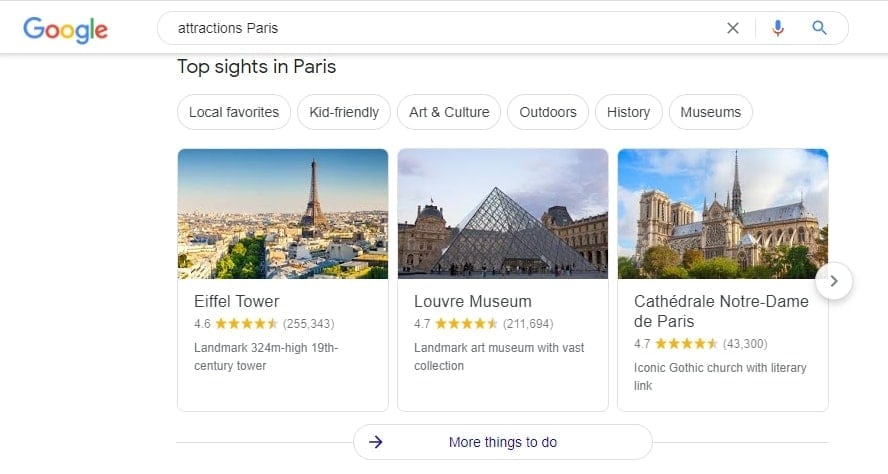The image captures a screenshot of a Google search results page focused on "attractions in Paris." In the upper left corner, the iconic multi-colored Google logo is clearly visible. Directly beneath it is the search bar with the phrase "attractions Paris" entered. Below the search bar, the results page primarily features black text on a white background.

The top section displays categorized rectangles highlighting various aspects of Parisian attractions, including "Local favorites," "Kid-friendly," "Art and Culture," "Outdoors," and "History and Museums."

Following these categories, three prominent images are showcased:

1. **Eiffel Tower**: Displayed with a clear picture of the Eiffel Tower against a sunny sky and bustling cityscape. The entry notes the Eiffel Tower's rating of 4.8 from 26,241 reviews. It is described as a landmark, standing at 324 meters high, and built in the 19th century.
   
2. **Louvre Museum**: Represented by a striking image of its iconic glass pyramid. The Louvre holds a 4.7 rating from 21,894 reviews and is recognized as a landmark art museum with an extensive collection.
   
3. **Cathedral Notre-Dame de Paris**: Shown with a beautiful photo of the cathedral against a semi-cloudy blue sky, and with some greenery in the foreground. This incredible Gothic church has an impressive 4.7 rating from 43,300 reviews and features an itinerary link.

Centered at the bottom of the screenshot, there is an additional rectangular box labeled "More things to do" in blue text, alongside a dark blue arrow pointing left.